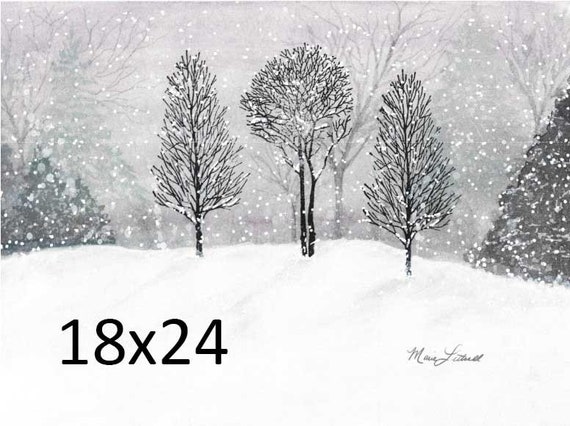This detailed black and white cartoon-style image captures a serene winter scene in a forest. Snow is gently falling, blanketing the ground and trees. In the center, there are several trees: some bare with just branches, and others evergreen with full pine needles. Mounds of snow surround these trees, adding to the peaceful atmosphere. The picture is horizontal and rectangular, with the dimensions "18 by 24" clearly labeled in bold black text on the bottom left corner. In the lower right corner, there's a gray signature of the artist who designed the image, although the name is not clearly legible. The combination of these elements creates a tranquil and snowy woodland landscape.